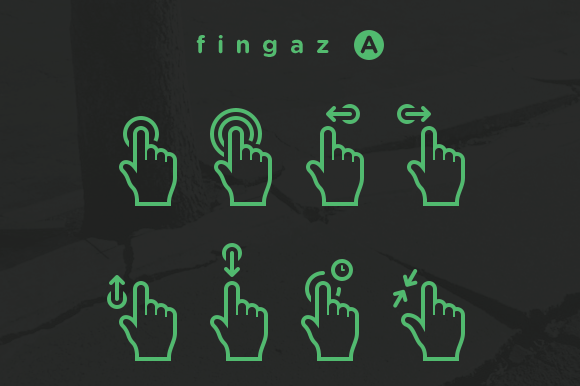This image is a tutorial poster entitled "FINGAZ." The title is centered at the top in medium green lowercase letters: "fingaz," followed by a green circle containing a black capital A. The background is a translucent black, revealing a faint, dark tree stump and cracked, snowy ground. Below the title, there are eight green hand icons arranged in two rows of four. Each icon is depicted with the pointer finger up and thumb out, suggesting various gestures commonly used on touch devices.

In the top row:
1. The first icon shows a finger pressing down with a semicircle around it.
2. The second icon displays a finger tapping twice with two semicircles.
3. The third icon features an arrow pointing left, indicating a swipe left gesture.
4. The fourth icon has an arrow pointing right, indicating a swipe right gesture.

In the bottom row:
1. The first icon shows an arrow pointing up, indicating a swipe up gesture.
2. The second icon features an arrow pointing down, indicating a swipe down gesture.
3. The third icon displays a semicircle around the pointer finger with a small clock, suggesting a long press.
4. The fourth icon shows two diagonal arrows pointing towards each other, indicating a pinch and zoom gesture.

The green icons are prominent against the dark background, emphasizing their instructional nature.